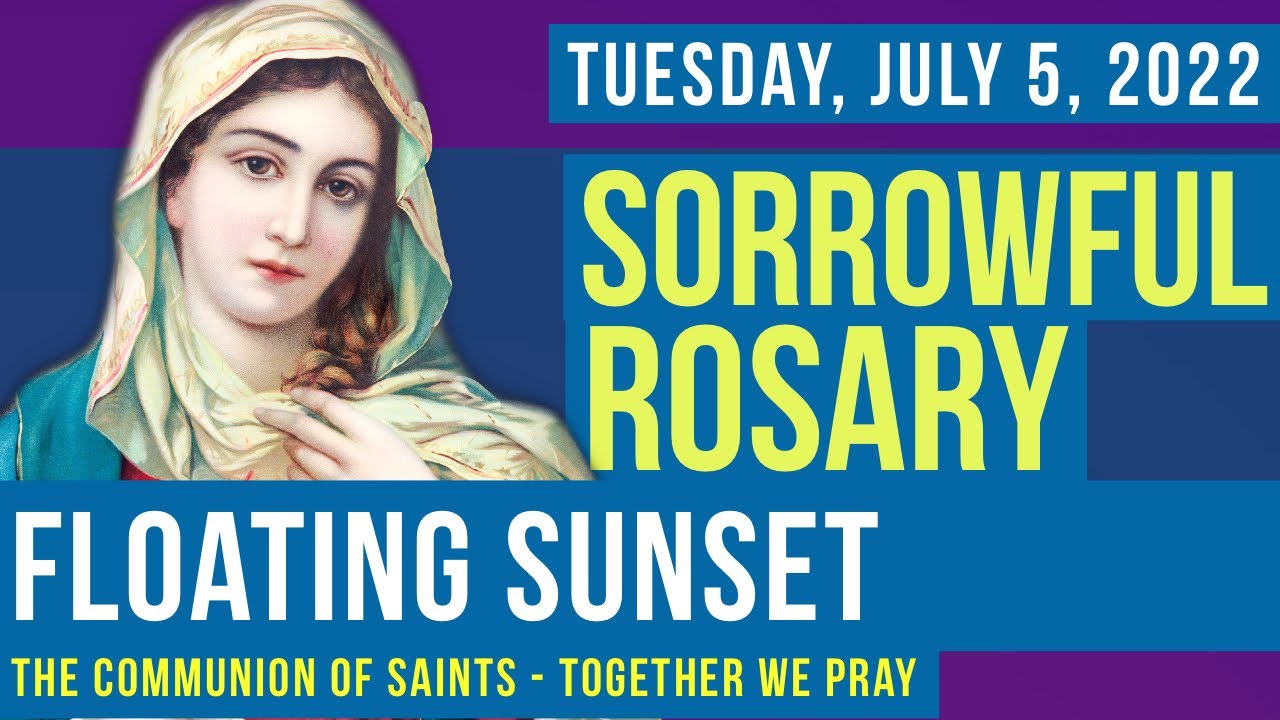A detailed poster features an image of a melancholy woman, possibly invoking Mary, adorned in a headscarf that drapes over her head and neck. She gazes directly at the viewer. The backdrop consists of vibrant, horizontal stripes transitioning from purple to shades of blue. She occupies the upper left corner of the image. Adjacent to her on the right, the date "Tuesday, July 5, 2022" is written in white text. Below it, the phrase "Sorrowful Rosary" is prominent in bold yellow letters. Further down the poster, blue labels successively contain the titles "Floating Sunset" in white and "The Communion of Saints, Together We Pray" in yellow.